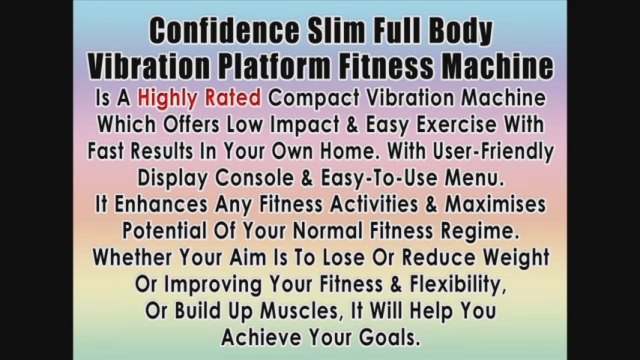The image is a colorful, rainbow-themed presentation with text printed in black. It showcases the "Confidence Slim Full Body Vibration Platform Fitness Machine," emphasizing its reputation as a highly-rated, compact device designed for home use. This machine is praised for offering low-impact, easy exercises that deliver fast results. It features a user-friendly display console and an easy-to-use menu. The text highlights how the machine can enhance any fitness regimen, helping users to lose weight, improve fitness and flexibility, or build muscles, ultimately assisting in achieving their fitness goals.